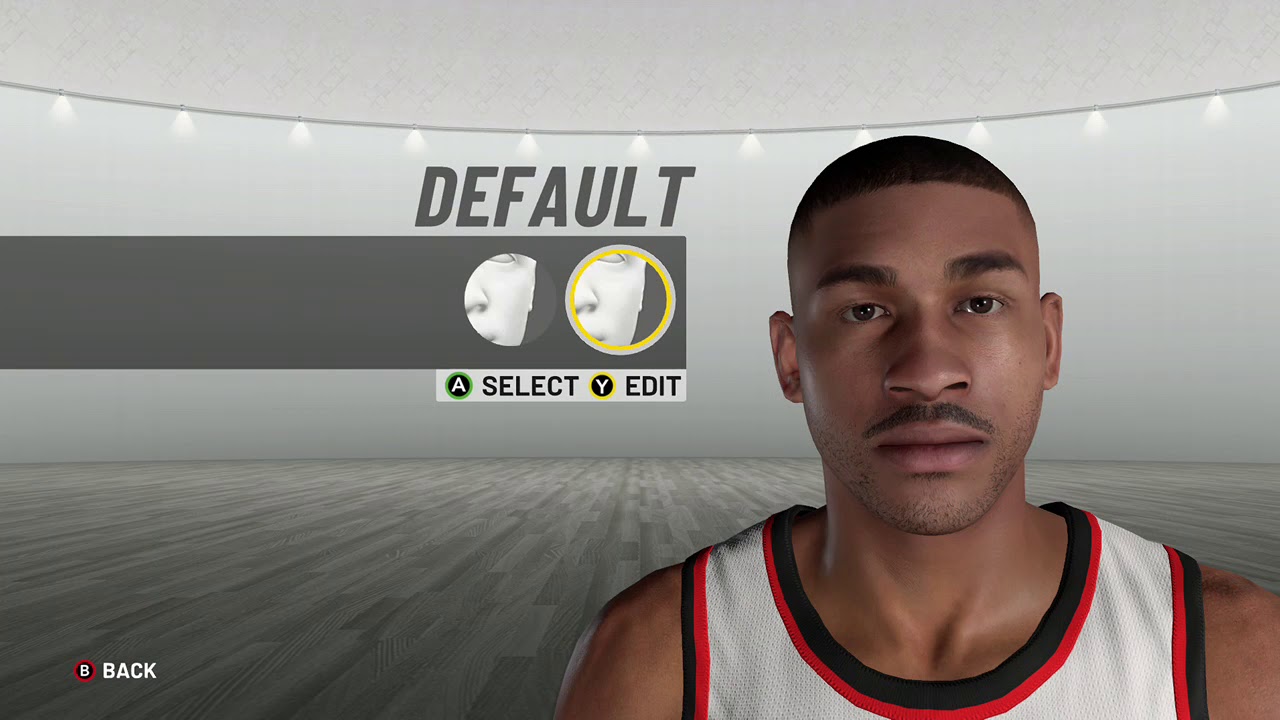The image is a screenshot from a sports video game, featuring a prominent close-up of a dark-skinned athlete with very short hair. The athlete, wearing a stylish white jersey with red and black trim and open sleeves, looks forward with a calm expression. In the background, the word "DEFAULTS" is displayed in large gray letters, positioned above a wide gray banner that offers two options. The banner includes facsimiles of a person's face without skin tone, with one of the options highlighted. Players can select options using the 'A' button or edit using the 'Y' button, indicated in the lower portion of the banner.

The setting is minimally detailed, with a plain screen in the background. The floor appears to be wooden, extending into the distance, and hanging above are simple light bulbs in a grayscale color scheme. In the lower right-hand corner, the letter 'B' is set inside a black circle with red edges, suggesting a control option within the game’s interface.

Overall, the image immerses the viewer in a scene that blends clear character visualization with a straightforward, user-friendly menu screen, characteristic of many sports video games.